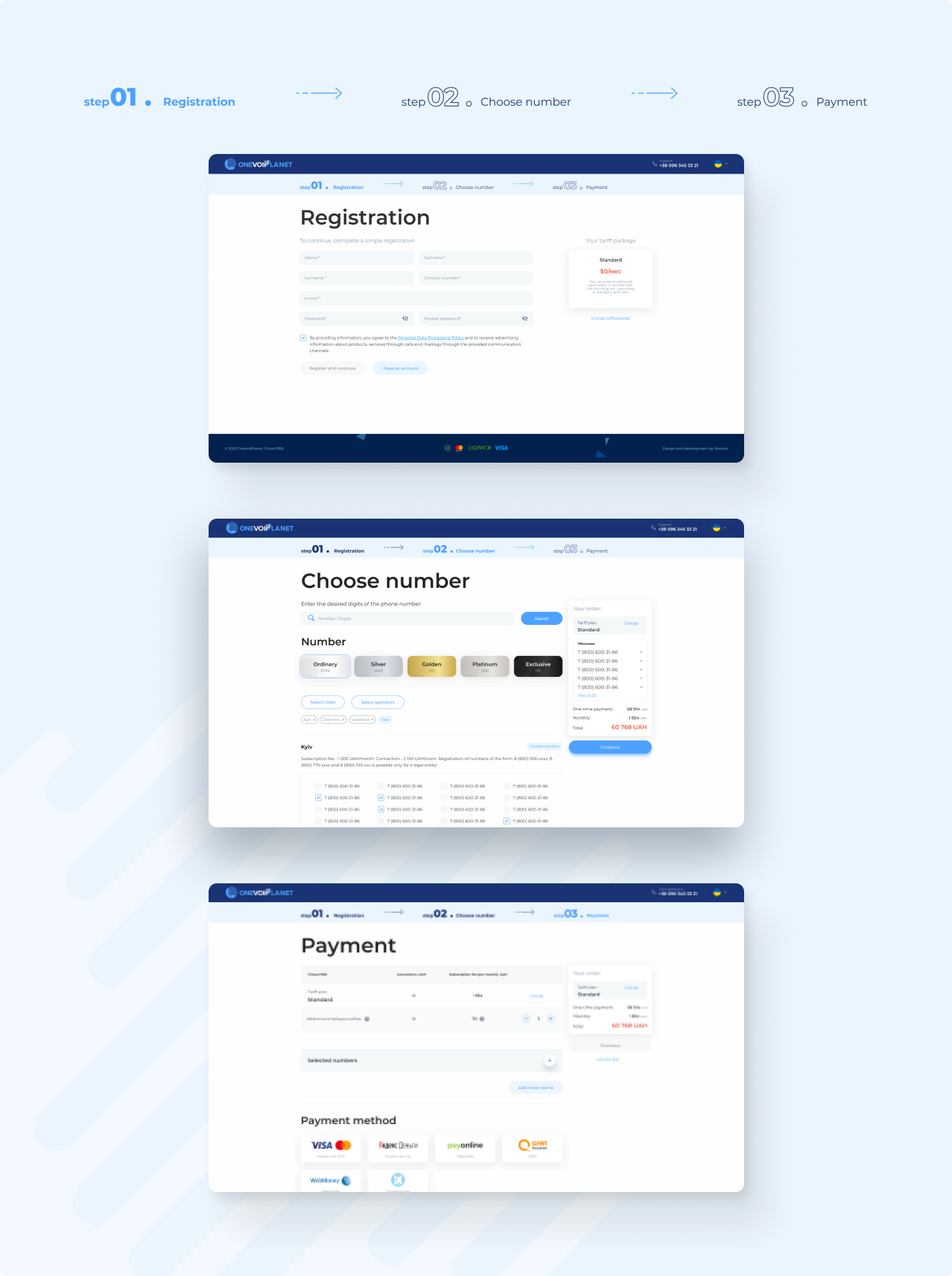This image depicts a three-step online registration process. The first step, titled "Registration," requires users to enter their personal details, such as their name and other pertinent information. The second step, labeled "Choose Number," involves selecting a specific number, although the details of this step are unclear due to the small size of the image. The third step, "Payment," features options for payment methods, including MasterCard and Visa, indicated by their logos. The compact size of the image makes it difficult to discern finer details despite attempts to zoom in.